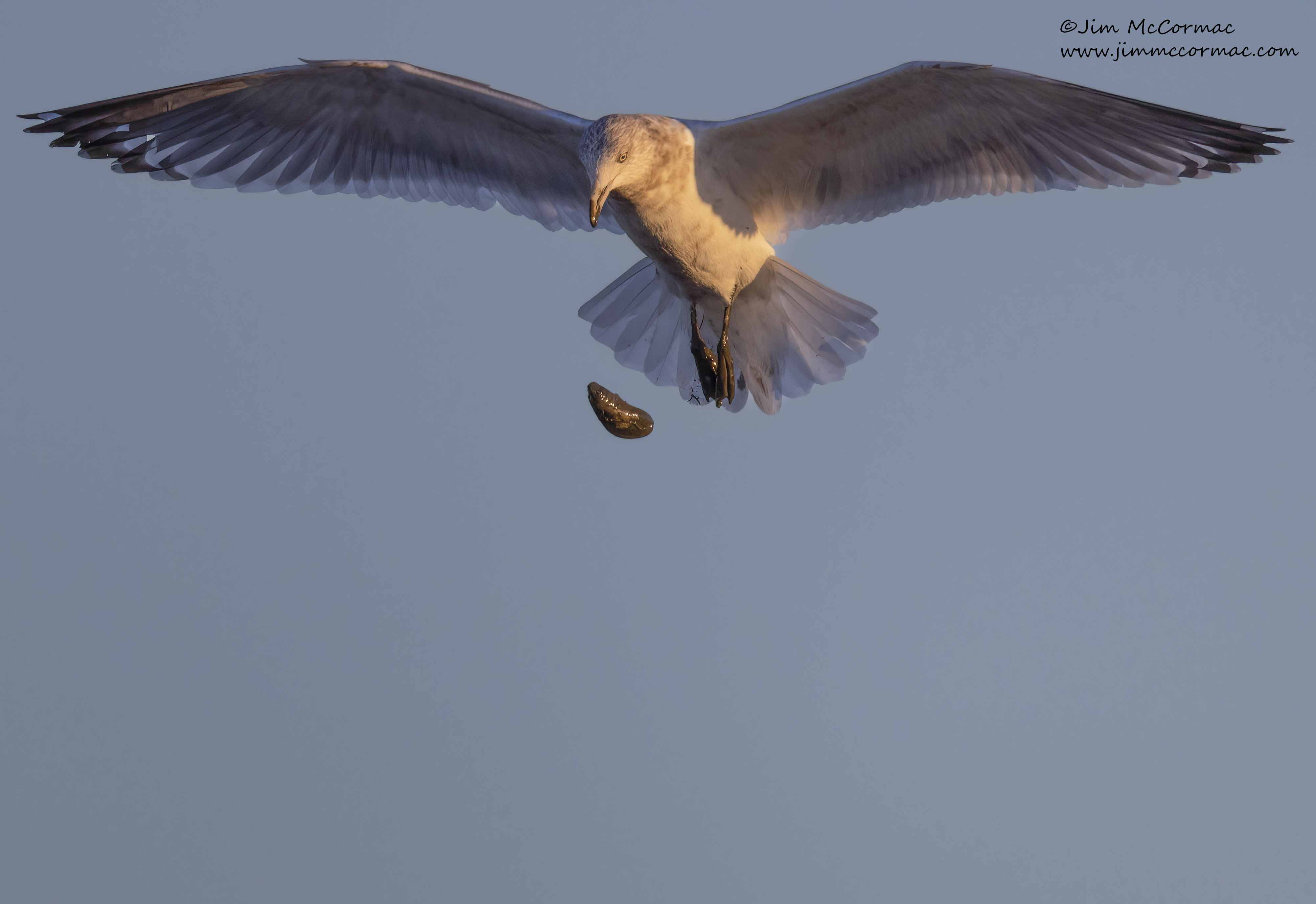The image captures a light cream-colored seagull with outstretched wings soaring through a bluish-gray sky. Its tail feathers form a slightly rounded semicircle as they fan out behind. The seagull's muddy brown talons dangle as it gazes intently downward at a muddy oyster or rock it has seemingly dropped. The bird's beak also carries traces of mud, hinting at a recent grip. Minimalistic in essence, the scene is accentuated by the inclusion of the text "at Jim McCormick" and "www.jimmccormick.com" in a semi-cursive font, positioned in the top-right corner of the image.